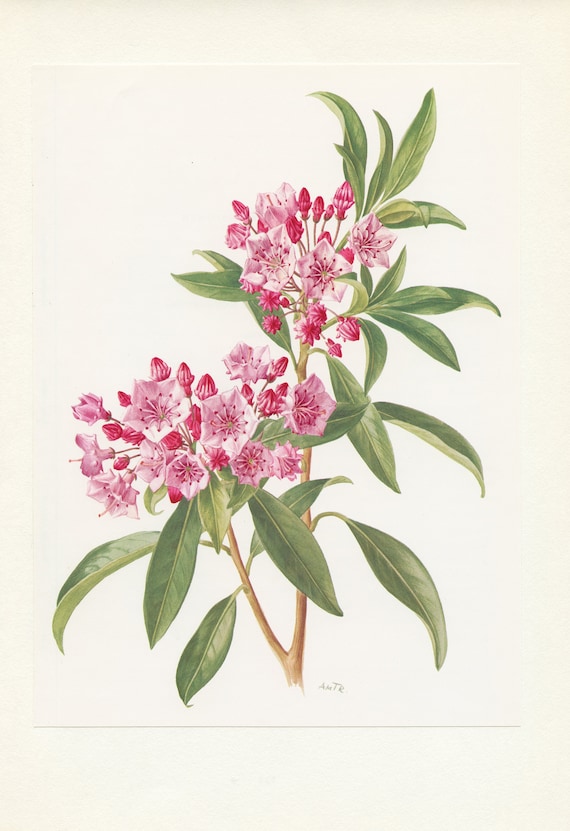This is an exquisite painting of a flowering plant rendered in a pastel or graphite style, characterized by high-quality detail. The plant features a brown stem that splits at the base into a Y or V shape. Sprouting from this stem are about a dozen individual green leaves. The tips of the two branches each boast a vibrant bloom of flowers, with petals in varying shades of pink, red, and purple, comprising around a dozen flowers in total. The art is set against a tan canvas, providing a subtle, harmonious background that enhances the plant's vivid colors. At the bottom of the stem, the artist's initials or signature can be faintly seen, though it is not easily readable. The image has an overall delicate and serene composition with no other objects or text, except for a faint black line at the bottom of the canvas.